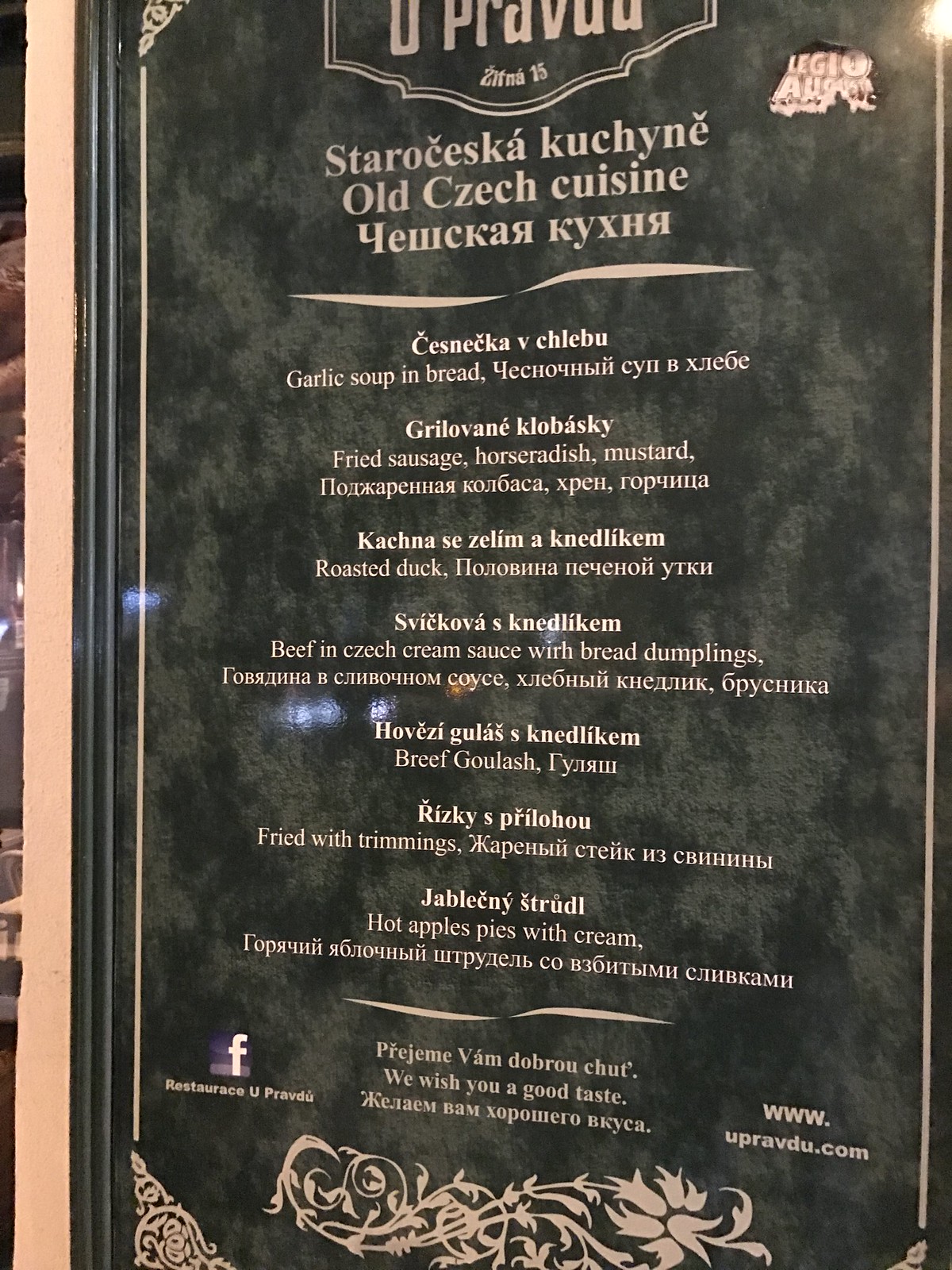This image showcases a menu board prominently displayed inside a restaurant. The main content of the menu is written in an Eastern European language, which appears to be either Russian or Czechoslovakian. The upper section of the menu features various dishes typical of Eastern European cuisine, including traditional items such as hot apple pies with cream, beef goulash, beef and cheese cream sauce with bread dumplings, roasted duck, and garlic soup served with bread.

In the lower right corner of the menu board, the website URL is provided: www.upravdu.com. Additionally, the lower left corner mentions "Restaurant of UPRAVDU," suggesting a link to their Facebook page for more information. The few English words interspersed within the menu offer a glimpse into the traditional dishes available, emphasizing the diversity and cultural richness of the restaurant's offerings. Overall, this menu represents a delightful culinary experience rooted in Eastern European traditions, likely situated near Russia or the former Czechoslovakia.